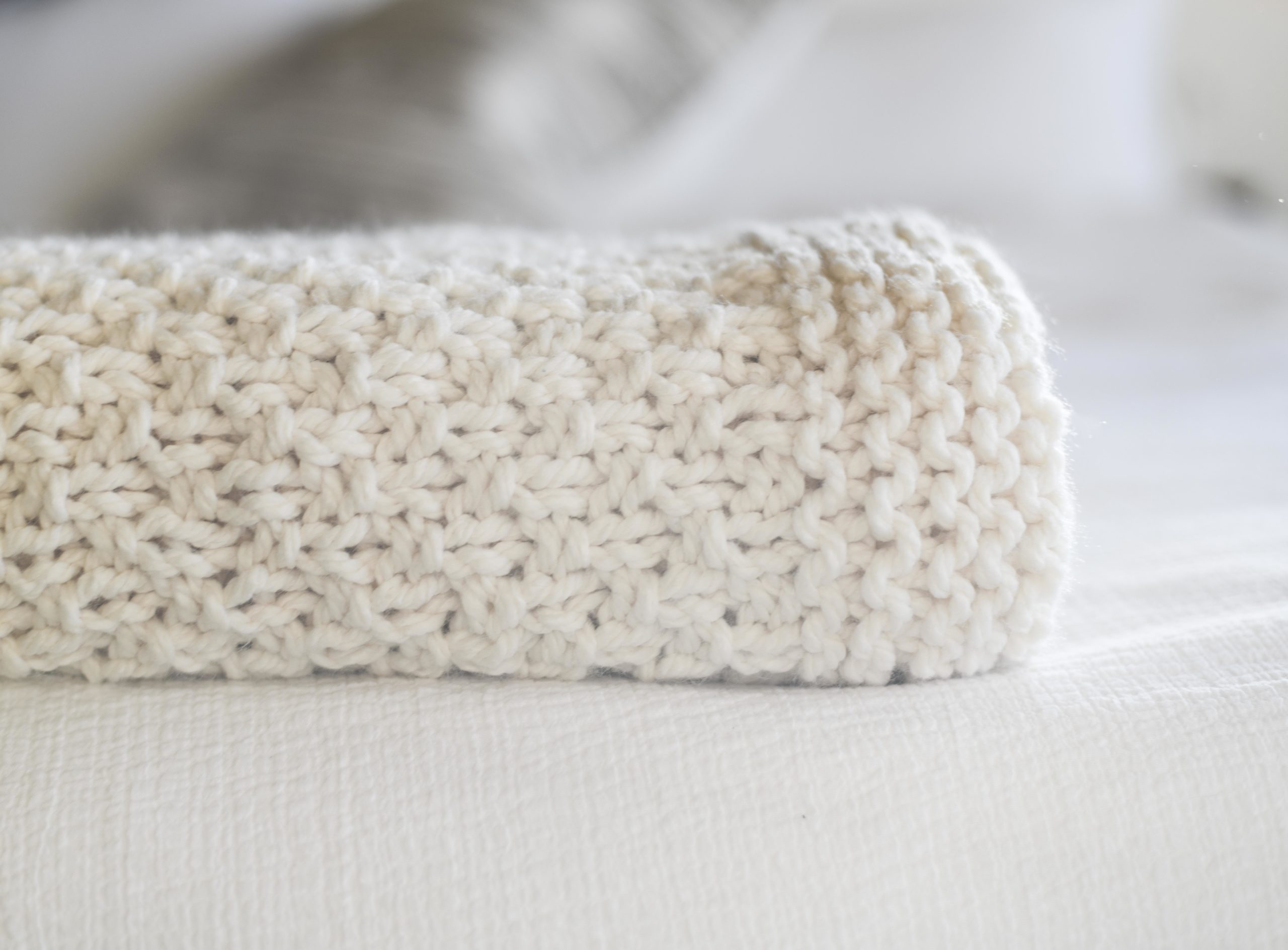This image features a close-up shot of a thick, chunky knitted blanket, folded neatly. The blanket appears to be made from very thick yarn, possibly some kind of animal yarn like alpaca wool. It has a white or off-white, somewhat creamy hue. The knitted texture and possibly crocheted details are prominently visible. The blanket is laid on a white surface, possibly a bed or a couch, surrounded by a blurry background with white and gray tones that offer a soft contrast to the knit. The image focuses primarily on the folded edge of the blanket, capturing its fluffy and cozy essence.